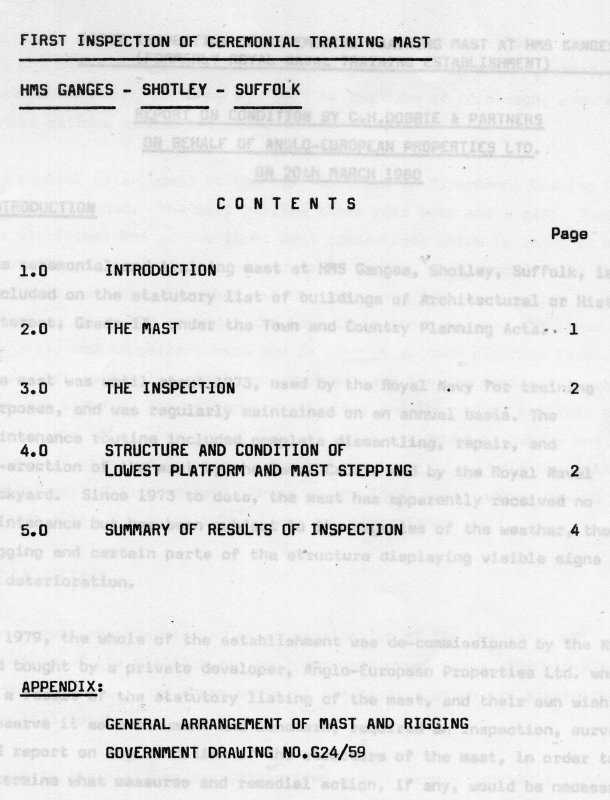The image is of a black and white document, specifically a table of contents from an official report. The title at the top reads "First Inspection of Ceremonial Training Mast," followed by "HMS Ganges, Shotley-Suffolk." The contents are outlined with the following sections: "1.0 Introduction," "2.0 The Mast," listed as being on Page 1; "3.0 The Inspection," on Page 2; "4.0 Structure and Condition of Lowest Platform and Mast Stepping," also on Page 2; and "5.0 Summary of Results of Inspection," on Page 4. At the bottom, there's an "Appendix" which mentions the "General Arrangement of Mast and Rigging Government Drawing Number G24/59." The formal text can be faintly seen showing through from the next page, although it is not readable. The document is devoid of images, focusing solely on the text in a formal font.